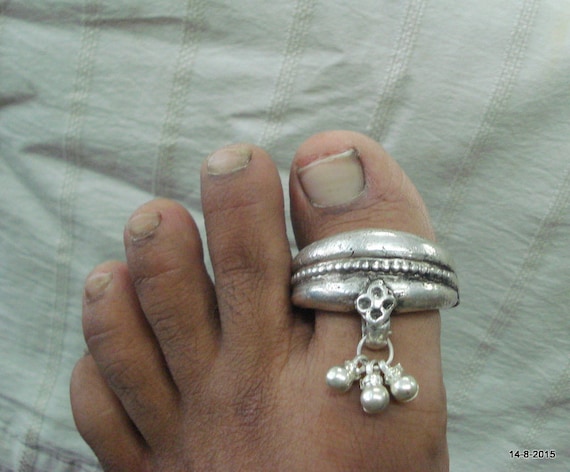The photograph, taken on August 14, 2015, is an amateur shot of the upper portion of someone's left foot, showcasing all five toes. The skin color of the foot is brown, and the toenails, including the cut but rough-looking big toenail, suggest a need for washing. The most distinct feature is a chunky silver or metallic toe ring on the big toe. This toe ring, a circular band with three small dangles, resembles either boxing gloves or ornaments but leans towards a less intricate, rather gaudy design. The foot rests against a backdrop of a bed or pillow, inferred to be green fabric with lines or possibly white or off-white bed sheets. This detailed composition highlights the foot and the toe ring against the textured background.